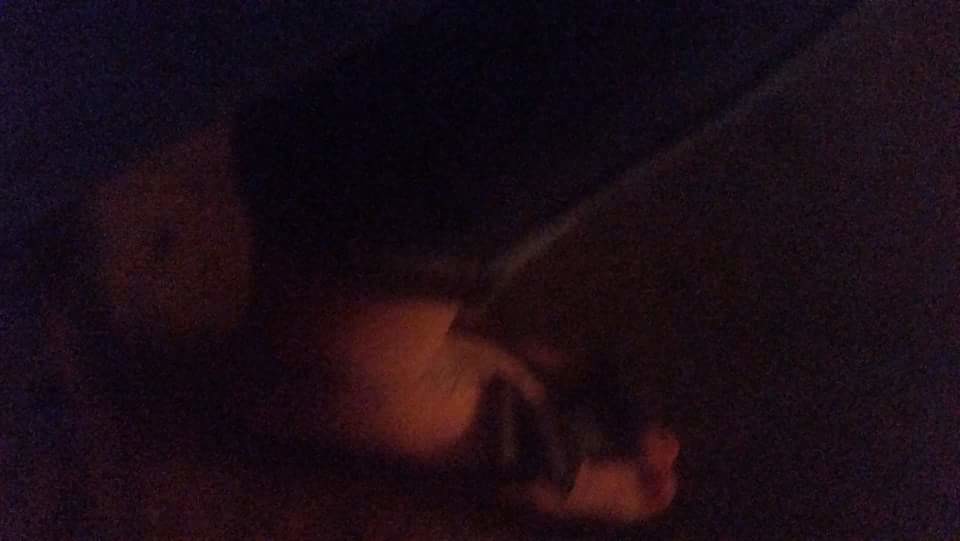In this horizontally-oriented, extremely dark, and blurry image taken late at night, the scene is heavily distorted and obscured, making object identification challenging. Predominantly, in the lower central part of the photograph, there is an indistinct whitish object that might be a pair of shoes or a piece of cloth, with an adjacent funnel-like structure. Extending from this object towards the upper right corner is a long, black, pipe-like element. This pipe-like feature seems to be held or connected by a reddish, rounded object, possibly resembling a hand or the top part of a flower. The upper left corner of the image is characterized by a black area, beneath which there is a light brown blur that transitions into an orangish-brown hue with a darker blur underneath. Additionally, a gray line-like object stretches from the upper right towards the center before cutting to the left. The photograph's poor lighting conditions, with minimal illumination, further complicate the visibility and detailed analysis of the scene.